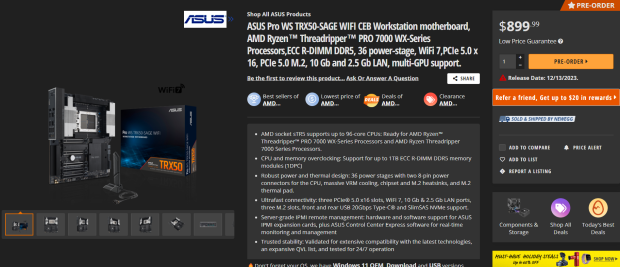In the image, there is an informational display for an ASUS computer product, presumably a computer tower available for purchase. The background of the page is entirely black, contrasting with the white text and other features layered on top. On the left side, the ASUS logo is prominently displayed at the top. 

Towards the center of the layout, albeit somewhat blurred, there is a diagram or illustration of what appears to be a computer tower. This may include internal components or an overview of the product's design, but the blurriness obscures finer details.

Dominating the central area, a clear white text outlines the model and specifications of the product: "ASUS Pro WS-TRX50 SAGE Wi-Fi CEB Workstation Motherboard AMD Ryzen Threadripper Pro 7000 WX Series Processors ECCR DIMM DDR5 36 Power Stage Wi-Fi 7." This long description details key features and compatibility options, suggesting the high-performance and professional-grade nature of this system, aimed at users requiring robust specifications. Overall, the page serves as a detailed specification sheet for a powerful ASUS workstation motherboard designed to support the latest AMD Ryzen Threadripper Pro 7000 WX series processors.